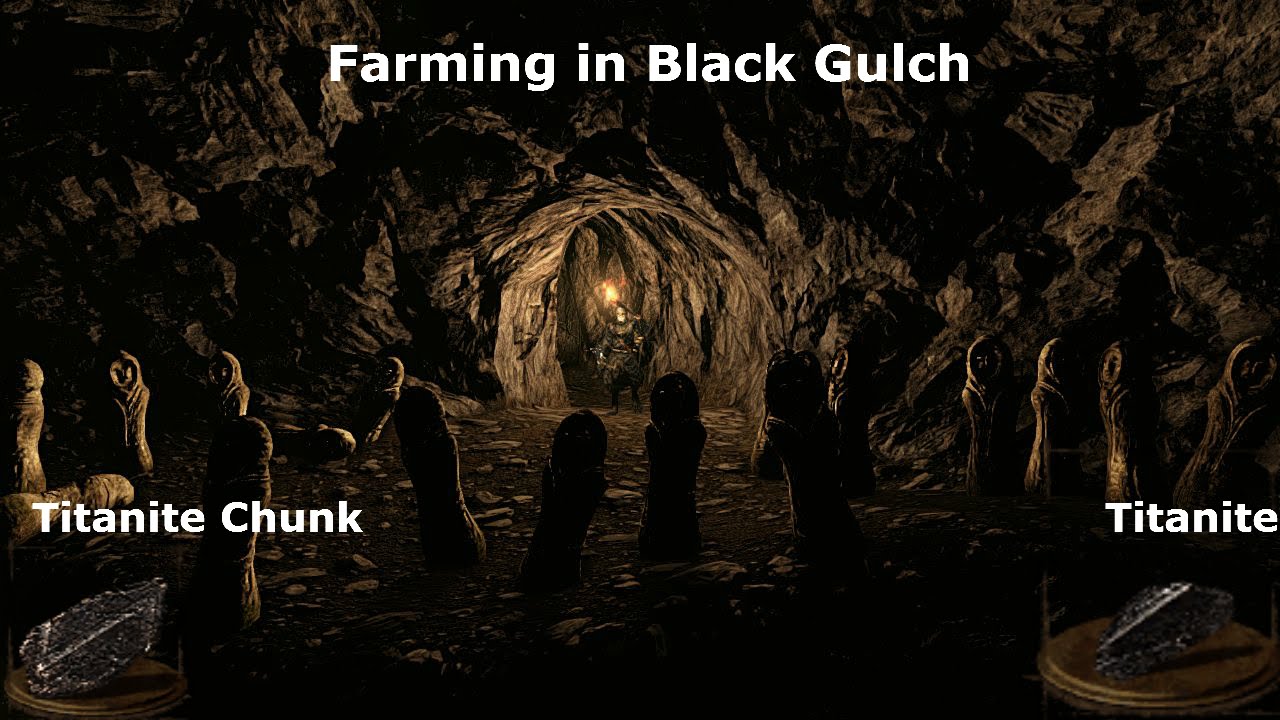The image is a highly detailed screenshot from an adventure video game, likely "Skyrim" or a similar title. The scene is set within a dimly-lit cave or cavern, featuring an entrance prominently in the far back. Just before this entrance, a humanoid figure stands armed and in a defensive stance. The top of the image is adorned with the title "Farming in Black Gulch" in uppercase for the initials. Toward the lower left corner, the text "Titanite Chunk" is visible, accompanied by an image depicting this element. Similarly, the text "Titanite" appears in the lower right corner, also with a representative image. The screenshot seems to serve as a guide, illustrating where to locate these materials and what they look like. Surrounding the central figure in the cave, a group of about 15 robed individuals can be noticed, possibly engaged in some ritualistic activity. The overall ambience is dark, accentuated by minimal lighting that highlights the elemental stones displayed on a platform or dias.